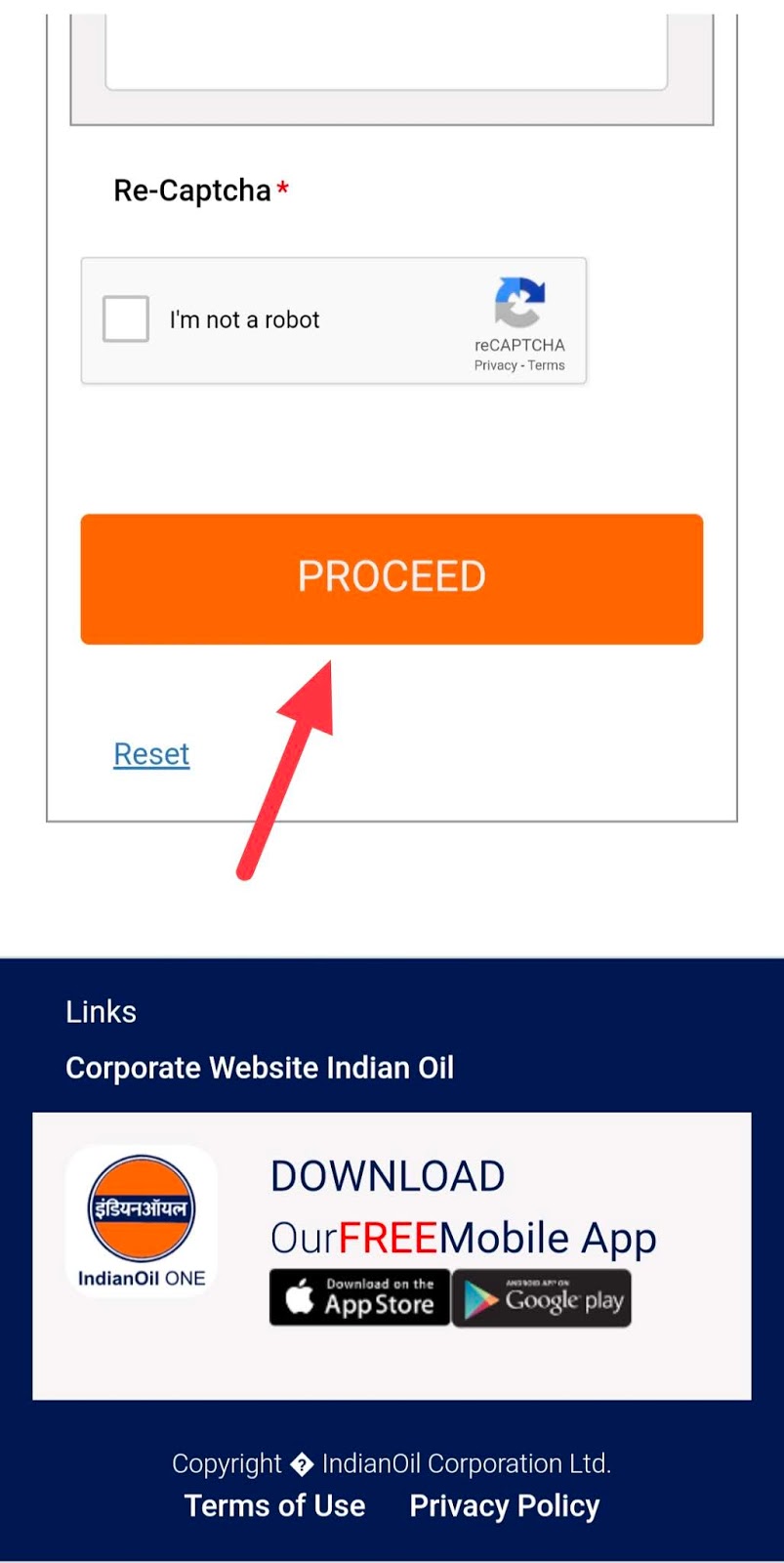The image displays a detailed user interface designed for a CAPTCHA verification process on a web page. 

At the top of the interface, there is a section resembling two overlapping pitchers, with the top one extending about two-thirds down the height of the bottom one. This section has a white background, decorated with two vertical black lines positioned about half an inch in from the left and right edges. These lines extend downwards to about an inch below the white section before turning horizontally towards the center. The lines meet towards the bottom, defining a bordered area within this section.

Below this white section, the interface transitions into a gray-bordered rectangle, which features the text "RE-CAPTCHA" in black, accompanied by a blue asterisk. Beneath it is a light blue rectangle stretching two-thirds across the width of the image. Inside this blue rectangle, there is a checkbox on the left side with the text "I'm not a robot" beside it, and the RE-CAPTCHA emblem with "RE-CAPTCHA" typed underneath.

About an inch below this area is an eye-catching orange tab that spans the entire width of the image. The tab contains bold, white, capitalized text stating "PROCEED." 

From the bottom-left corner of this tab, a red arrow points upwards from just outside the border, adding emphasis. To its left, in the bottom-left corner of the interface, the word "RESET" appears in blue, underlined for emphasis.

There is an inch-wide gap below this section, leading to a lower dark blue border. At the center of this border is a white rectangle that occupies about half of the width. Within this white area, the word "LINKS" is positioned at the top-left corner followed by "Corporate Website" and "Indian Oil" below it. In the white area, an orange circle is present on the left side with the text "Indian Oil" next to it. To the right of this, bold, all-capital text reads "DOWNLOAD OUR FREE MOBILE APP," with icons for the Apple App Store and Google Play located beneath.

At the bottom-most part of the interface, outside the white rectangle, the text "COPYRIGHT INDIAN OIL CORPORATION LTD." is situated, followed by "TERMS OF USE" and "PRIVACY POLICY."